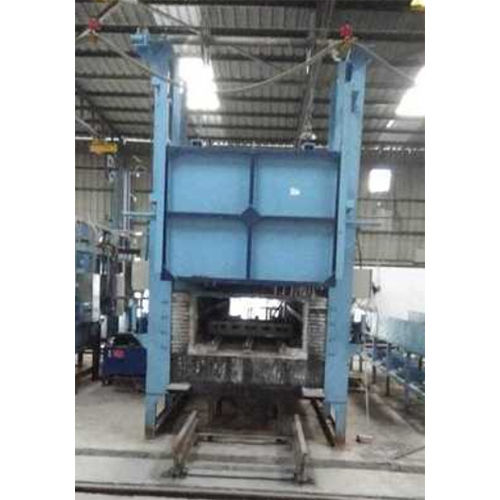Inside a bustling warehouse, a large industrial machine dominates the scene. This machine, encased in light blue metal with dark blue trim, stands prominently on beams, creating an open, tunnel-like space beneath it highlighted in black and gray hues. It appears to be mounted on a track, suggesting it can move forward and backward, although its specific purpose remains unclear. The interior of the machine seems to be lined with concrete bricks, giving it the appearance of a kiln, yet its function is ambiguous, potentially related to fabrication, shredding, or another industrial process. Surrounding the machine, the warehouse hosts various other machinery and metal fixtures. To the left, rows of shelving and a blue dumpster are visible, while to the right, more tables and shelves store additional concrete bricks. The floor is made of white concrete cement, and fluorescent lights illuminate the space from above, with gray cables hanging both from the machine and the ceiling. In the background, there is an open section leading either outside or to another room, further adding to the industrial atmosphere.